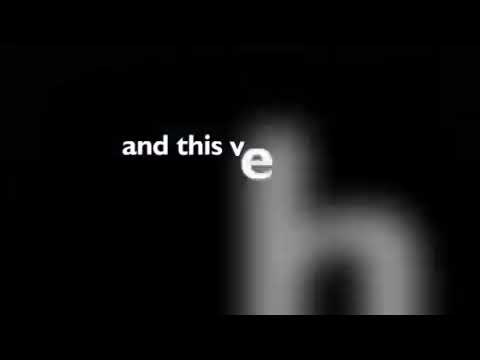The small, slightly wide rectangular image features a digital logo or advertisement set against a completely black background, with a distinct black strip running along the bottom. Positioned in the lower right quadrant of the image is a very blurry and large object resembling a lowercase letter 'h.' Towards the middle left of the image, in thick white lowercase font, are the words "and this," arranged horizontally. Adjacent to the word "this," is the letter 'v' in the same white font, followed by a slightly larger and somewhat fuzzy lowercase letter 'e', situated just below and to the right of the 'v'. The blurry 'h' occupies much of the lower right portion of the image, contributing to a sense of incompleteness and out-of-focus elements in that area. The complete image is clearly framed with a black border at the bottom.